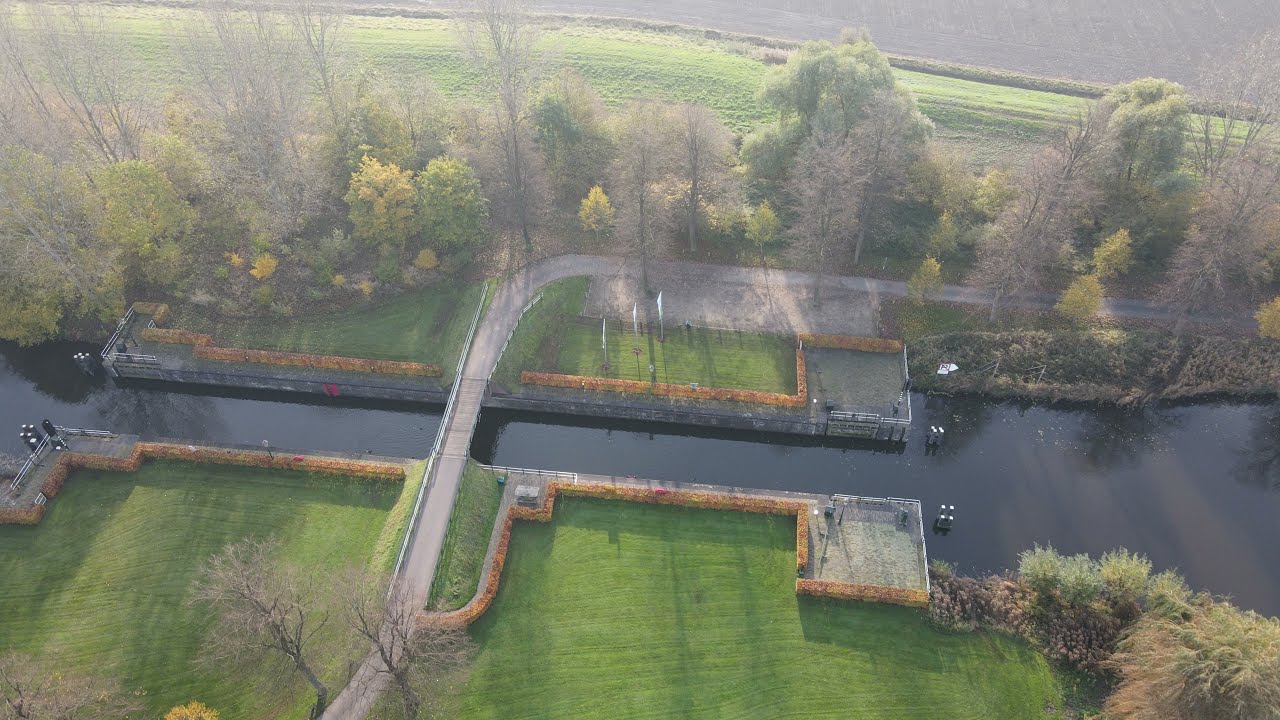The image is an overhead view of a narrow canal with brown, murky water that widens as it moves to the right side of the picture. A small bridge spans this canal, with white barriers on either side, and posts sticking out of the water alongside this waterway. Surrounding the canal are areas of short cut grass, and an embankment lined with shrubs and flowers that have turned yellow and contain reddish hues. 

Adjacent to the bridge, a road enters from the center right of the image before turning left and then downwards to cross the bridge at the bottom of the picture. Bordering the road are tall trees, featuring a mix of green, yellow, and bare, leafless branches, indicating a seasonal transition, likely springtime. Behind this stretch of trees lies a large, open, gray area that is indistinct, possibly another water body or a parking lot. The backdrop is lush with expansive fields and scattered green vegetation, giving the entire scene a vibrant, natural atmosphere.